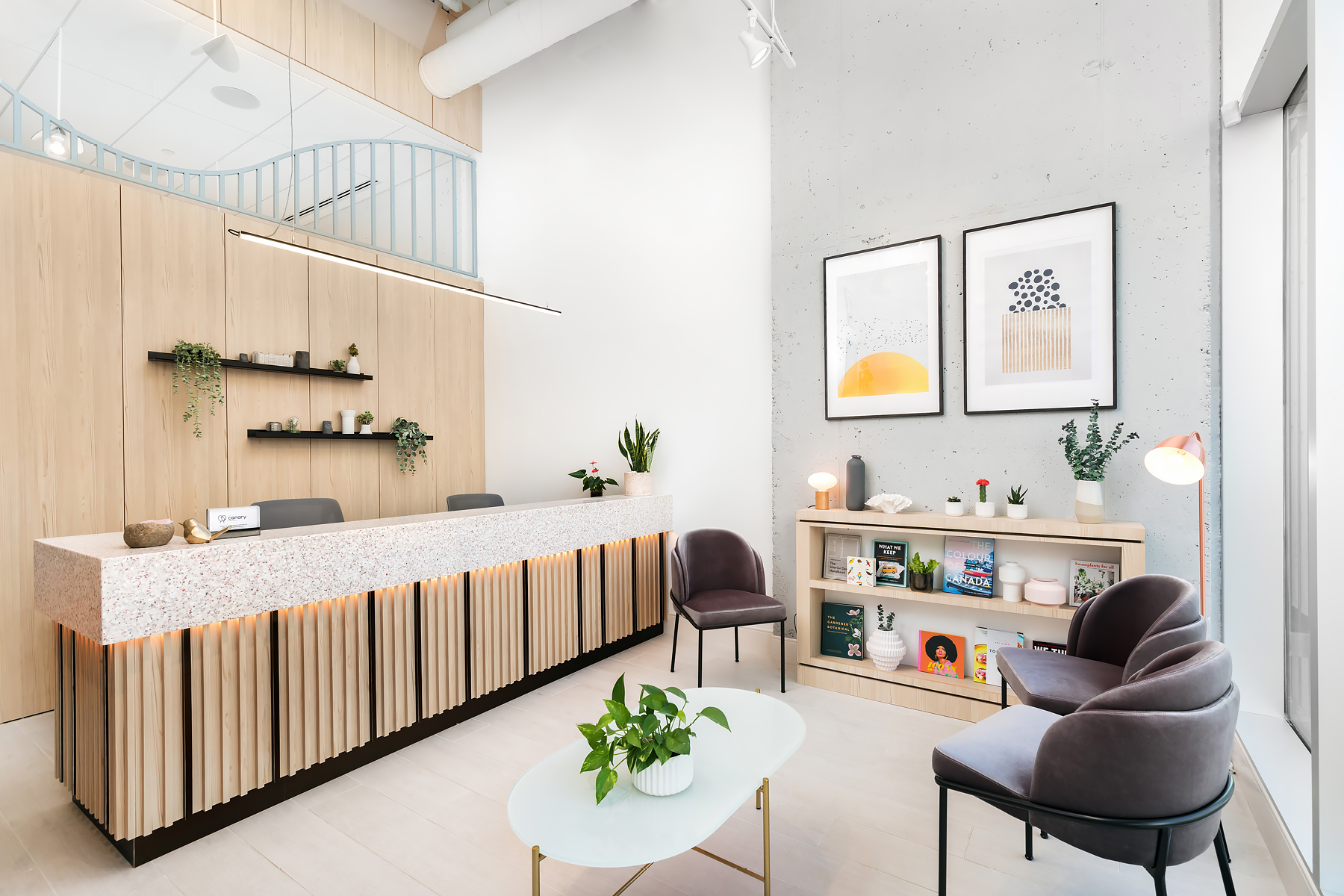This realistic, modern waiting room, likely part of a spa or medical office, features a harmonious blend of functionality and aesthetics. The focal point is a prominent front desk with a sleek, wide, granite countertop adorned with a variety of plants, a rustic bowl, a metal bird figurine, and an unreadable placard. Behind the desk, two shelves showcase a mix of greenery and decorative items, contributing to the room's serene ambiance.

The room also includes a set of three medium-backed chairs with large, curved, gray cushions on metal frames, positioned around a small, white coffee table with gold metal legs and a rounded rectangular top. A potted plant in a white pot sits at the table's center, adding a touch of nature. The walls are painted in a mix of white, light tan, and gray accents, and are adorned with two pieces of art—one depicting half of a sun and the other featuring abstract lines and dots. 

Additional touches include a bookcase with magazines and plants, a corner lamp, and some decorative knickknacks. The setting is well-lit with a long, hanging fluorescent light and promotes a calm, inviting atmosphere with its neutral color palette and cozy furnishings.